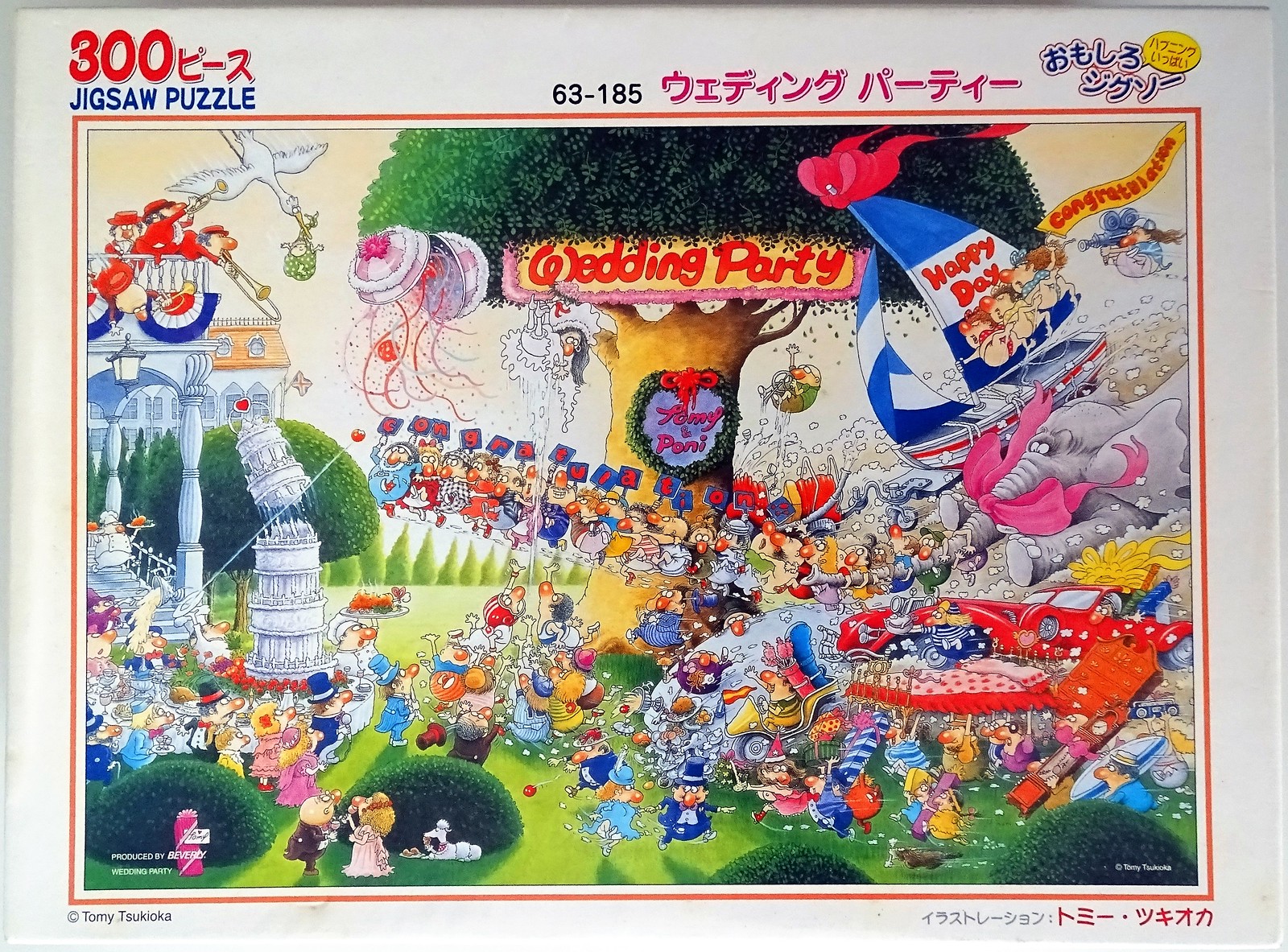The box cover of this 300-piece jigsaw puzzle is detailed and colorful, featuring a light white or light gray border. In the top left corner, "300" is prominently displayed in red letters, accompanied by symbols to its right and "jigsaw puzzle" written underneath in blue. Centered towards the top is the code "63-185," with adjacent purple Asian characters and additional text in the upper right corner with a yellow circle containing red writing.

The main image showcases an extravagant and intricate wedding party scene set outdoors, possibly in a courtyard. In the center rises a large, umbrella-shaped tree adorned with a red sign that reads "wedding party" among its green leaves. Beneath the sign, streamers flutter in the air, and the tree trunk is decorated with a green wreath.

A lively procession crosses the scene from left to right, featuring small characters and people, some carrying balloons, a large sailboat with "happy day" inscribed, and an elephant wearing a pink scarf entering from the right. Below this animated display is a verdant grassy area crowded with tiny figures, a towering cake with its top askew, and several green shrubs.

In the foreground, a dog lies beside a couple hidden behind a bush, characters and animals mingle, and green hedges lead to a large house in the background. Musicians play on a balcony, and a crane or stork carrying something flies in from the upper left. The intricate and vibrant scene is packed with delightful details, creating a bustling, celebratory atmosphere. At the bottom left of the white border, there is an illegible name in black writing, while the bottom right features black and red Asian characters.